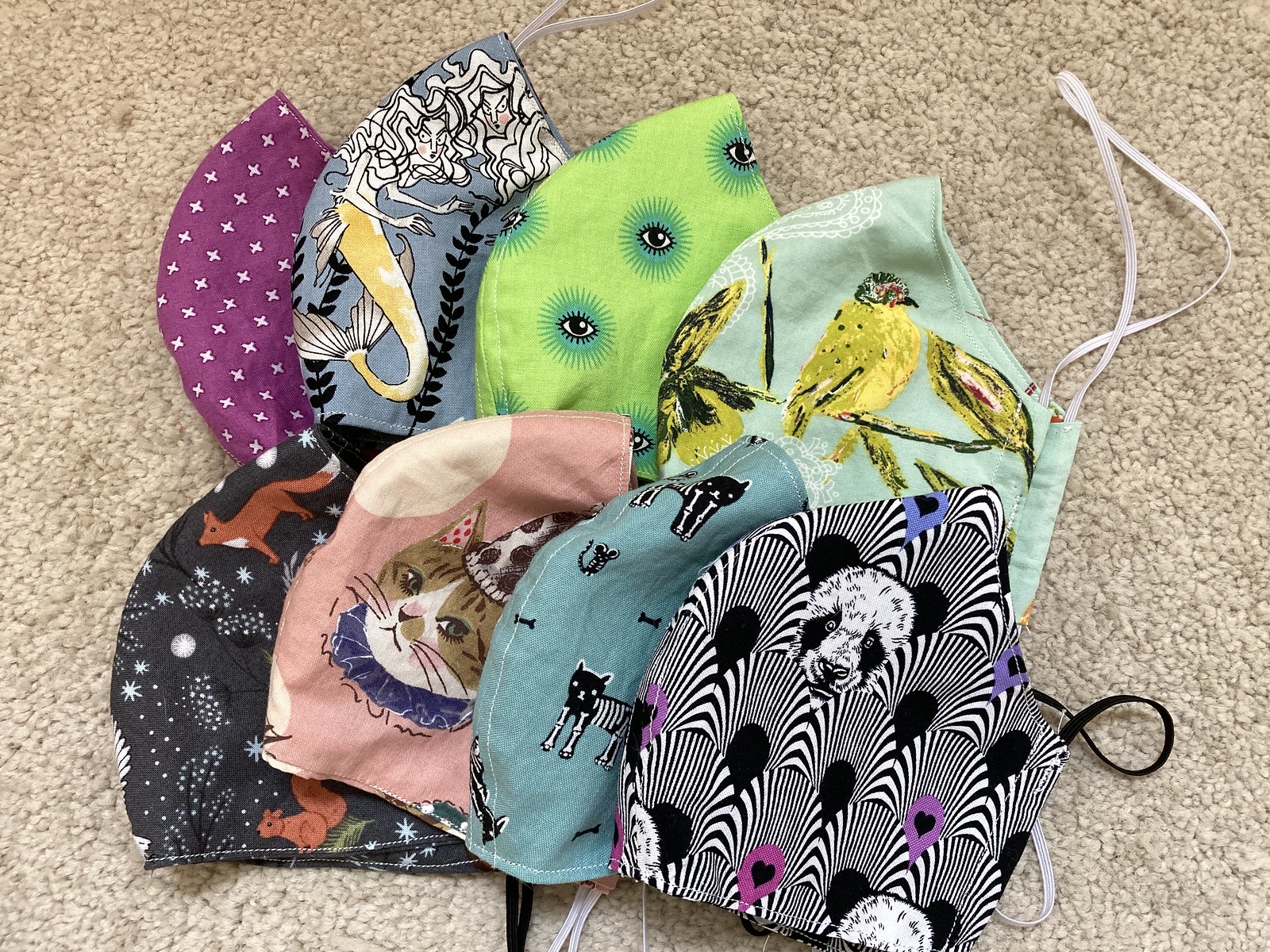The image showcases an array of eight custom fabric face masks displayed on a beige carpet. These masks are intricately arranged in a slightly overlapping, fanned-out manner, revealing their unique and diverse designs. Each mask features a different patterned fabric, harmonizing a blend of both bold and subtle artistic expressions. The masks include various themes such as:

1. A blue mask adorned with a whimsical mermaid with flowing white hair and a yellow tail.
2. A black mask featuring vivid red and white foxes standing amongst clusters of white stars.
3. A green mask patterned with eyeball designs encased in starburst shapes.
4. Another green mask displaying delicate images of yellow birds perched atop twigs.
5. A mask with a black-and-white design illustrating a panda bear camouflaged in swirling patterns.
6. A light blue mask showcasing a cat in a black-and-white polka-dotted party hat with a dark blue neckcloth.
7. A purple mask embellished with four-pointed star motifs.
8. A gray mask depicting a bird perched on a twig against a starry backdrop. 

Each mask's artistic pattern creates a visually striking and diverse collection, all elegantly laid out on the low-pile carpet, depicting a moment captured during the COVID era.